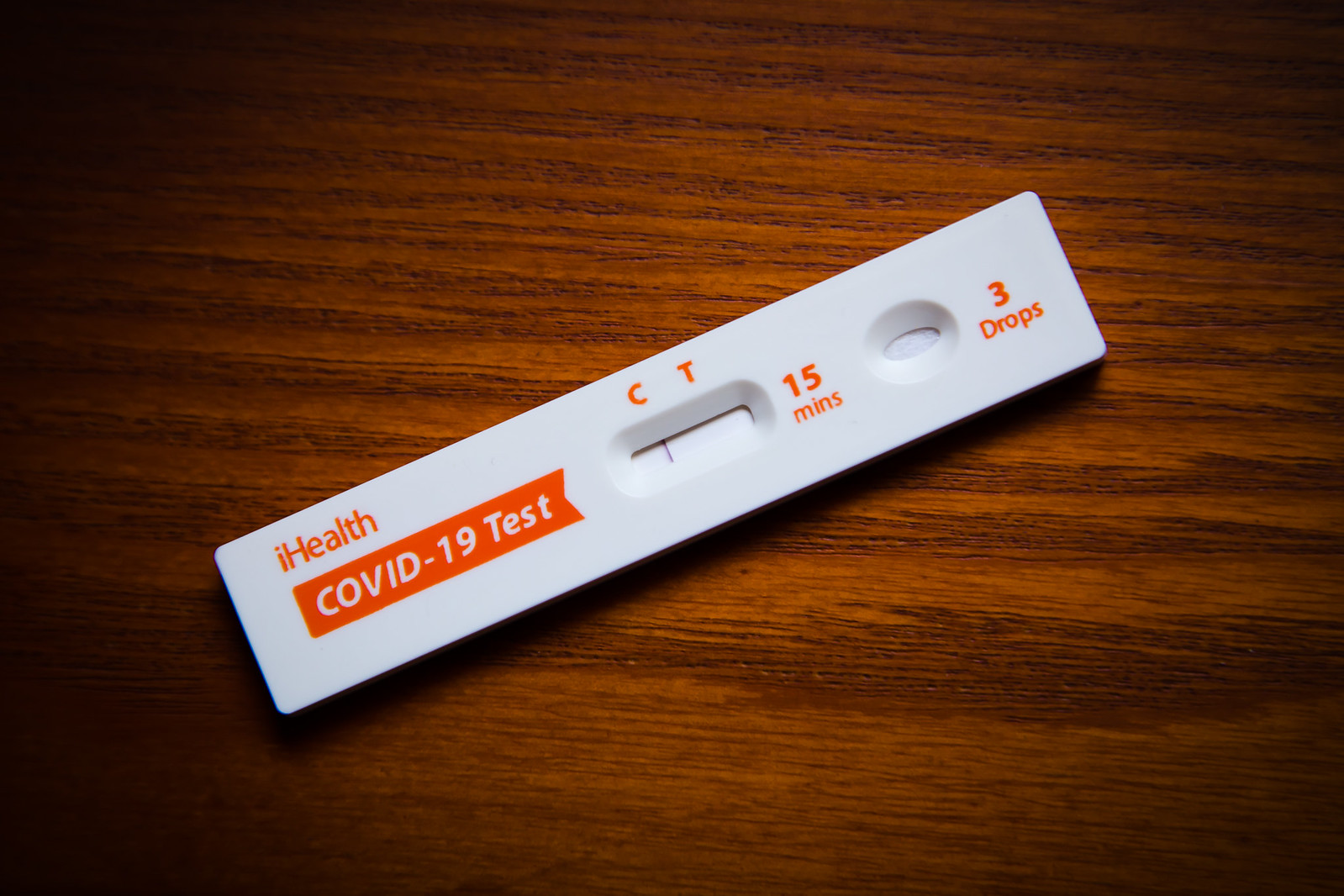The image features a COVID-19 test kit placed on a woodgrain table. The test is positioned flat against the table, angled so that the bottom edge is lower than the right side. The test kit is a thin, rectangular device with a white background. On the upper left corner, "iHealth" is printed in orange, with a lowercase "i" and an uppercase "H". Immediately below this, within an orange banner, the words "COVID-19 Test" are displayed in white letters.

In the central portion of the test is an oval-shaped window where the results appear. The letters "C" and "T" are printed in orange next to this window, with a black line under the "C," indicating the control line for test validity. To the right, the duration "15 minutes" is written in orange. Next to this is another oval window, and further right, the instructions "3 drops" are printed in orange letters, indicating the number of drops of liquid to be applied for the test.